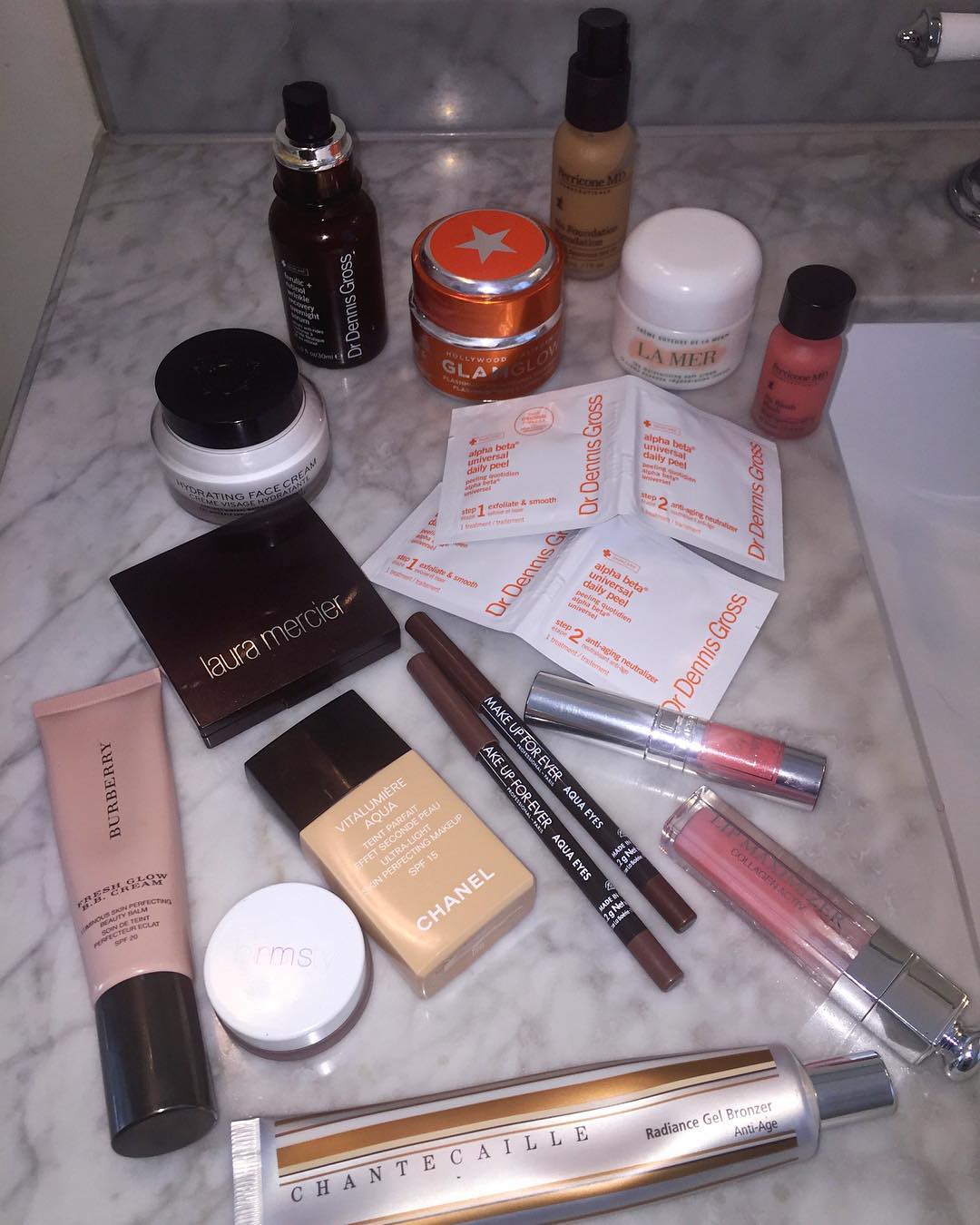The image showcases a cluttered sink area adorned with various bottles, containers, and papers. The sink, with a white and light grey textured design, forms the primary setting of the scene, with its white basin visible on the right side. The wall in the top left corner is also white, maintaining the clean aesthetic of the space.

Centrally featured is a round red container boasting a white star and red circles on its lid, with the label "Hollywood Clark Lowe." To its left stands a dark brown glass bottle with a white cap and a silver ring, labeled "Dr. Dennis Cross" in white text. This bottle also has a black sticker with white text.

Below the glass bottle, a container with a black cap and marked "Morating Face Cream" in black text is visible. Adjacent to this, a dark brown and red square box displays the name "Laura Messia."

Further down, a distinctive black-and-brown rectangular container is labeled "Willow Smell, Aqua, Chanel," though some text appears blurry. Another container below is white with a brown base, labeled "RMS."

In the bottom right corner, a plastic tube with the word "Blueberry" written in black text lies horizontally, topped with a white cap. Positioned at the bottom is another tube facing right, inscribed with "Chante Kiley, Reggie, and Shirley Brown's Auntie H."

Among the disarray, additional makeup products are visible at the front, including items labeled "Makeup Forever." There are also two pencils present, one of which is labeled "Dr. Dennis Cross" with white text and orange accents.